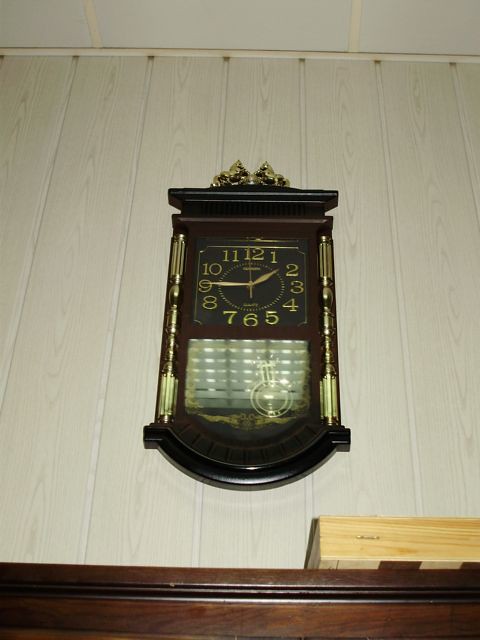This photograph captures an upward-looking view of a wall, which exhibits vertical slats of white-painted wood, creating a light wood grain appearance. The ceiling above the wall is trimmed with white and includes drop tiles. Centrally mounted on the wall is an old-style clock, characterized by a dark brown wood outline and a vertical rectangular body that tapers into a rounded bottom. The clock face is black, featuring gold numbers and hands, encased by gold detailing running down the sides. Above the clock, there is a gold decorative object. Below the clock face, a clear glass section reflects window shades with light filtering through. At the very bottom of the photograph, there is a dark brown shelf, partially visible, with a thick book resting on it; the brown wood grain of the book is discernible, as are its white pages. The overall image highlights the intricate detailing and reflective elements of the clock against the backdrop of the white paneled wall.